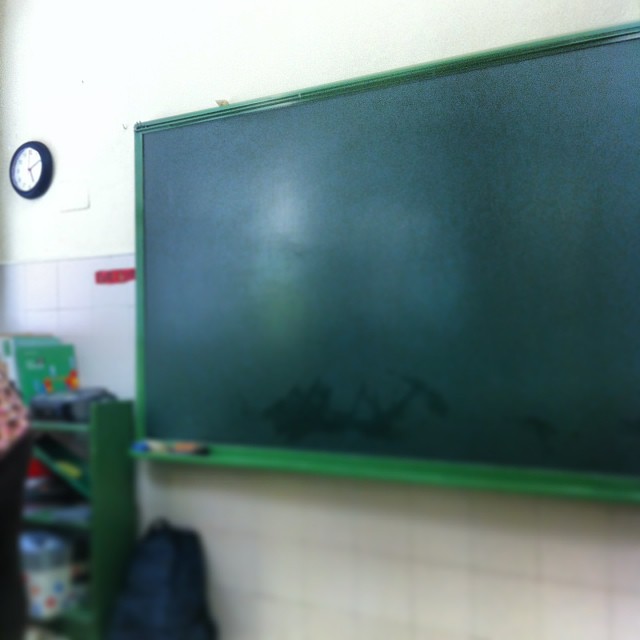In this classroom setting image, a large green chalkboard dominates the scene, positioned toward the center and extending to the right-hand side. The chalkboard is worn, appearing black in the central area, with additional blur at its bottom left corner suggesting objects resting on its lower rim. In the top left corner of the image, a white wall covers nearly half of the upper section. A black circular clock is affixed to this wall, with its red and black hands approximately indicating the times of five minutes past two. Below the white wall, the surface transitions into a gray block wall, extending downward.

On the far left side, partially within the frame, a green cubby is visible. Peeking out from the left, there also seems to be the back of a human figure, with accents of oranges and yellows scattered nearby. These colorful items appear propped up against the block wall beside the cubby, though their exact nature remains indistinct. This scene captures the characteristic details of a typical classroom environment, with an amalgamation of educational tools and everyday paraphernalia.